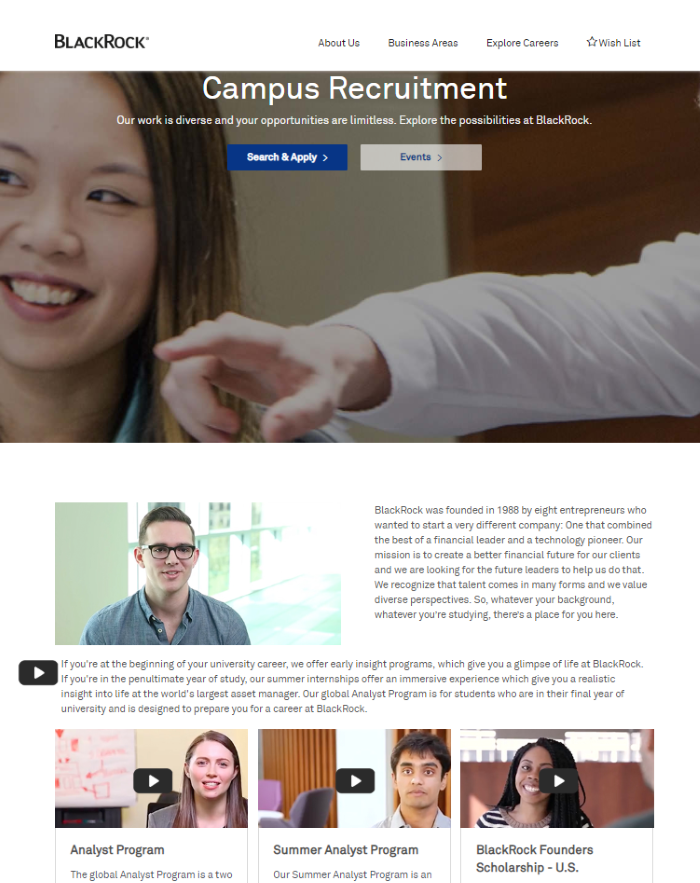The screenshot captures a segment of BlackRock's careers page focused on campus recruitment. At the very top, a prominent header displays the text "Campus Recruitment" over a large image occupying roughly one-third of the page. Underneath the header, a brief description reads, "Our work is diverse and your opportunities are limitless. Explore the possibilities of BlackRock," inviting prospective candidates to consider a career with the firm.

The BlackRock logo is positioned in the top left corner, while the top right corner houses a navigation menu with options: About Us, Business Areas, Explore Careers, and Wishlist, all rendered in black text. Notably, Wishlist is accompanied by a small star icon to its left.

The middle and lower sections of the page feature several thumbnail images from videos that highlight employee experiences and internship opportunities at BlackRock. Toward the bottom, three specific video thumbnails are displayed, each with a title: "Analyst Program," "Summer Analyst Program," and "BlackRock Founders Scholarship US." These videos likely offer insights into the respective programs and scholarships available to candidates.